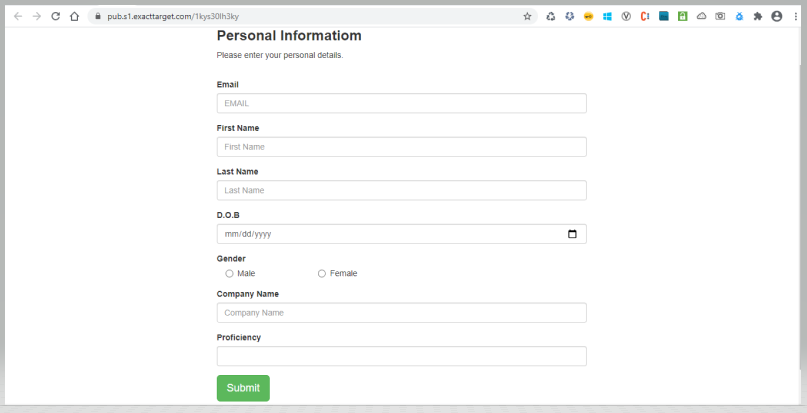The image depicts a webpage from ExactTarget's website, designed for customizing or adding details to a personal profile in 'light mode'. The background is white with black text, creating a clean and minimalist aesthetic. At the top of the page is the web address, "pubs1.exacttarget.com/[key code]", indicating a secure, personalized section of the site.

In the browser window, several icons are visible on the right side, representing various apps that the user can access. This specific page is titled "Personal Information" and features a prompt requesting the user to "Please enter your personal details." 

Currently, the form is empty. It includes input fields for Email, First Name, Last Name, and Date of Birth, formatted in the US style (MM/DD/YYYY). Additional fields for Gender (with options for Male and Female), Company Name, and Proficiency are also present. 

Beneath the form is a prominent green 'Submit' button, with the text 'Submit' displayed in white, inviting the user to input their details and finalize the process.